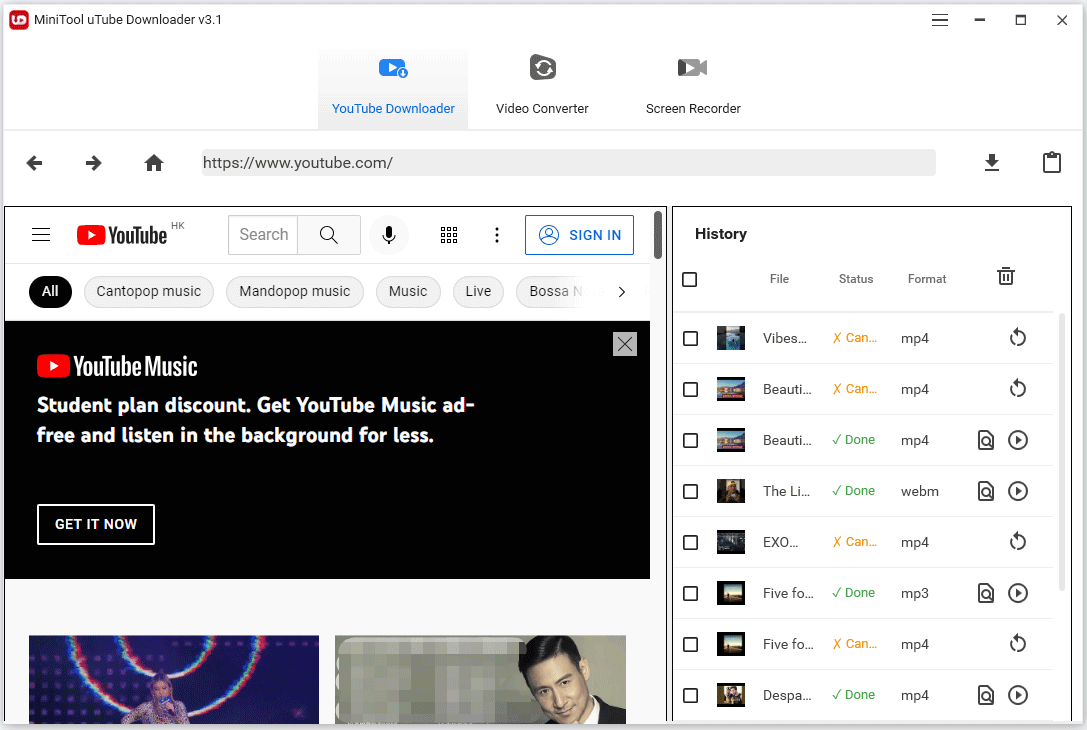### Detailed Caption for MiniTool YouTube Downloader Screenshot

The screenshot is from a YouTube interface, displayed within the MiniTool YouTube Downloader Version 3.1 software. The interface has a white background with a variety of text colors.

At the top of the screenshot, the text "MiniTool YouTube Downloader version 3.1" is prominently displayed alongside a small red graphic and several icons. The "YouTube Downloader" option is highlighted in blue, accompanied by additional icons such as a play button, a video converter, a manila folder with arrows, and a screen recorder. Nearby, there's a small camera icon with a play button on it.

Moving down the interface, there are gray back and forward arrows, a house icon, and a web address bar showing "YouTube.com". To the right of the address bar, there are icons including a downward download arrow and a clipboard icon.

Below this section, two images are shown side by side. The first image replicates the YouTube home screen, featuring the familiar elements: the YouTube logo with its play button, a search box, a microphone icon, several square icons, and a sign-in button. Categories displayed include "Canto Pop Music," "Mando Pop Music," "Music Live," and "Bossa Nova."

There's also a black promotional box on YouTube's home screen with text in white that reads "YouTube Music Student Plan Discount. Get YouTube Music ad-free and listen in the background for less," with a "Get It Now" button and a corner "X" for closing the box.

In this promotional section, two images appear: one featuring a woman with long hair dressed in a long sleeve shirt against a black background, and the other showing a man with black hair, a white collared shirt, and a black jacket against a tan background. Part of his image looks privacy-pixelated, and he is also partly juxtaposed against a white background containing various file formats and icons.

The second screen section of the downloader interface lists detailed file information. Headings include "History," "File Status," and "Format." Each file entry is accompanied by icons like a trash can, check boxes, small status indicators (orange for canceled, green for done), and file formats such as mp4, mp3, and webm. Additional icons include arrows, magnifying glasses, and documents, each corresponding to different file entries and statuses.